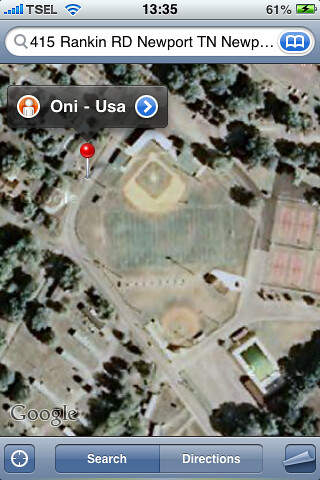The image is a cell phone screenshot featuring a map app, likely Google Maps, with the typical interface elements visible at the top, such as the time (13:35), battery percentage (61%), and a carrier indicator (possibly T-Cell). The search bar at the top displays the address "415 Rankin RD, Newport, TN," with the abbreviation "NEWP..." hinting at the full name of the town. The main focus of the map is an aerial view of a sports complex surrounded by trees, centered around a baseball field with the home plate facing north. The field appears primarily green, although some grass in the outfield looks dead. A road encircles the entire complex, providing access. Additionally, there’s a red pin marking a specific location on a roadway, and several characteristic map elements are visible, including the light gray "Google" watermark with a white border, a compass on a light blue strip, and search and directions buttons. An icon labeled "ONI USA" appears with a person's silhouette inside an orange circle. Towards the bottom right of the map view, there's an old-style peeling page effect reminiscent of earlier iPhone map interfaces.